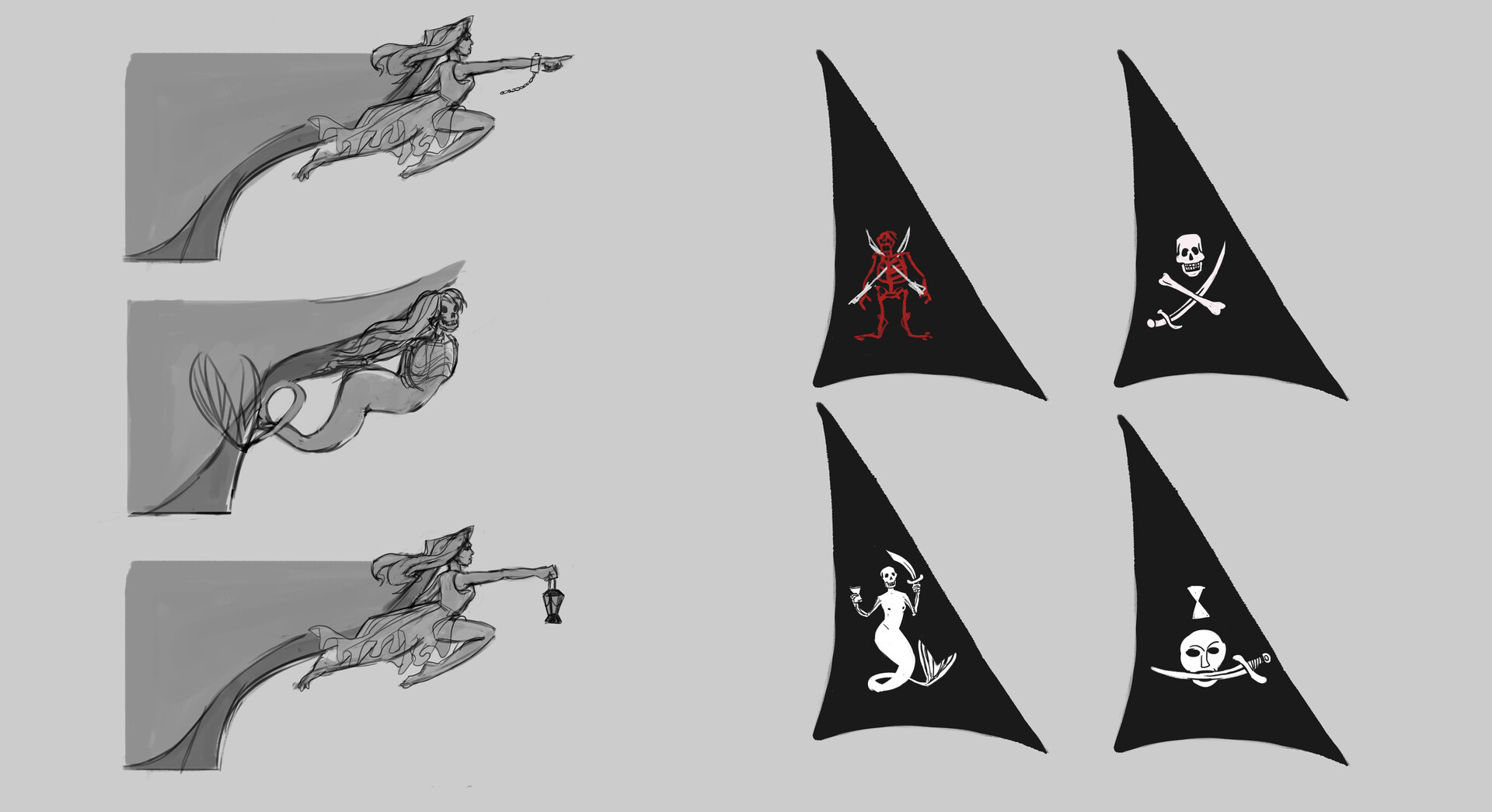The image features a detailed, artistic design set against a grey background. On the right-hand side, four triangular black pennants are arranged in a grid. From top to bottom and left to right, the pennants display: a red skeleton with knives crossed, a skull with a sword and a bone forming an "X," a mermaid wielding a saber in her left hand, and a human face in silhouette clenching a saber in its mouth. Each insignia is dark-themed, evoking a pirate or nautical motif.

On the left-hand side, there are three intricately hand-drawn figures resembling ship mastheads, commonly found on pirate vessels for good luck. The top figure is a woman pointing into the distance with her right hand, appearing as if in flight. The middle figure is a skeletal mermaid, her lower body curving elegantly backwards. The bottom figure depicts a woman holding a lantern in her right hand, seemingly to guide the way.

Overall, the composition of red, black, white, and grey elements creates a cohesive pirate-themed design, blending skulls, mermaids, and nautical imagery in a captivating, hand-drawn style.